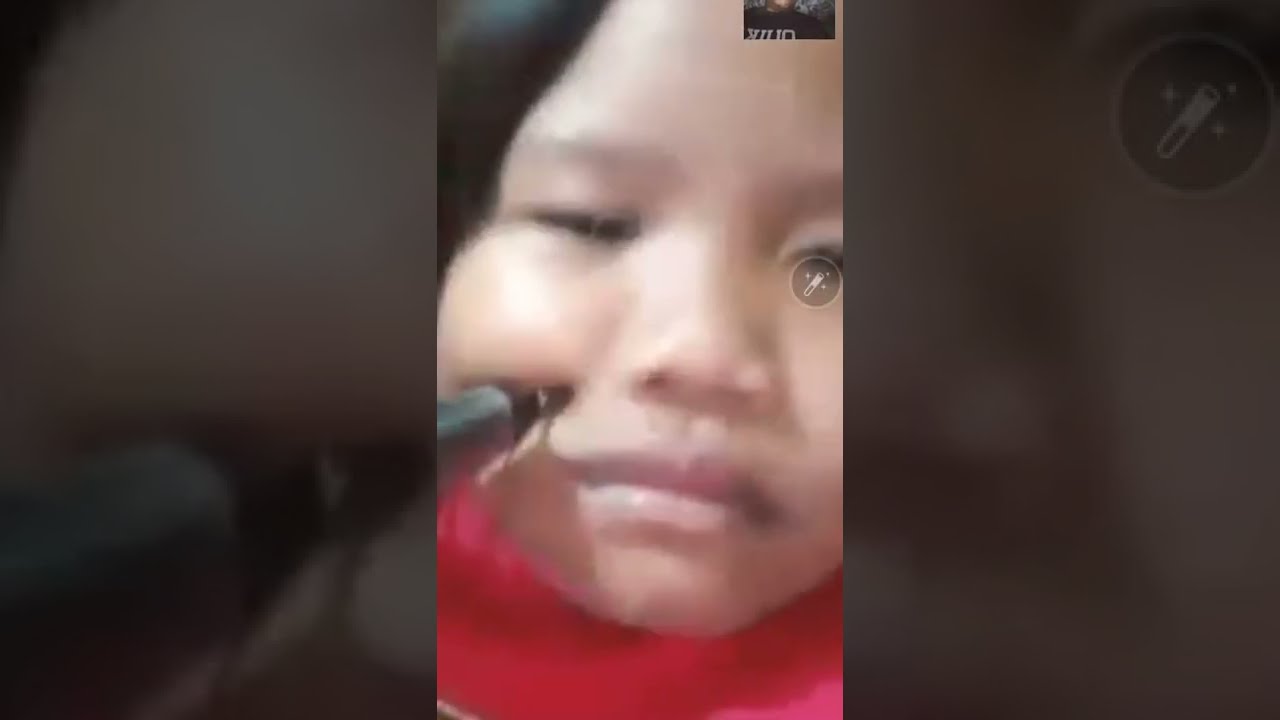This image is a detailed composite divided into three sections. The central section displays a vertically-oriented, somewhat blurry photograph of a young Asian child, likely a girl, who is intently focusing on something. She has light brown skin, black hair, and is wearing a reddish-pink shirt. Her face appears expressionless and slightly tired as she looks towards the viewer.

The child holds a silver pen with a black tip against her left cheek, near her mouth. The left and right sections of the image are magnified close-ups of the child’s face and the pen, with both sections appearing darker and more detailed than the central image. In these side sections, the close-up of her cheek and mouth are particularly prominent.

Additionally, overlaying the image are digital editing tools: above the child’s right eye (the eye on the left in the image) is a small grayed-out circle featuring an icon of a wand with magical sparkles, suggesting a filter or editing option. The top right corner contains another icon, and there is a small square in the upper left corner. The overall composition suggests a digital editing scenario, with the lighter central image flanked by two detailed, darker magnifications.